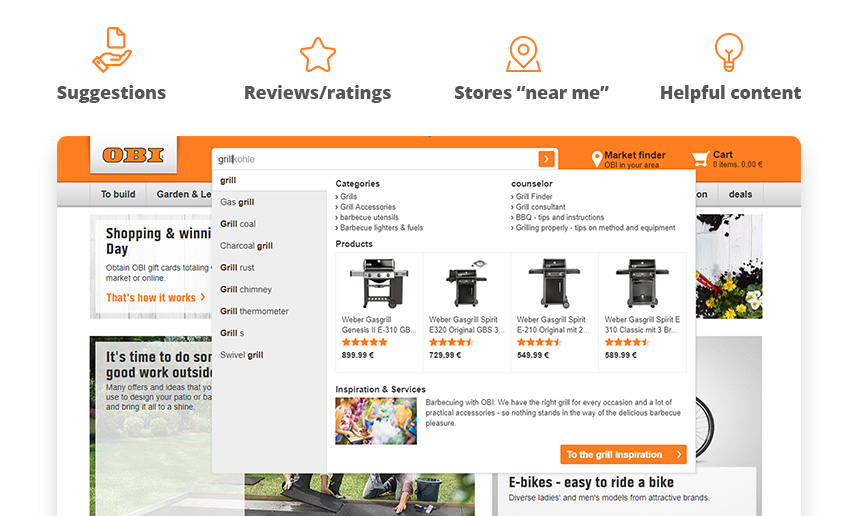This image displays a screenshot from an online shop called "Obi" (O-B-I). In the search bar of the website, a query has been made, and a dropdown window appears showcasing various grill options. The dropdown lists four different grills, each with its price in euros, ranging from €549 to €899, indicating that this shop is likely based in Europe. 

Above the product listings, there are categories and a section titled "Counselor," though its specific function isn't clear. Beneath the grill products, another section offers "Inspiration and Services," prominently featuring a headline that reads "Barbecuing with Obi." The text assures customers they have the right grill for every occasion, along with practical accessories, to ensure nothing stands in the way of a delightful barbecue experience. 

The grills featured appear to be high-end and premium, catering to those looking for quality barbecuing equipment.